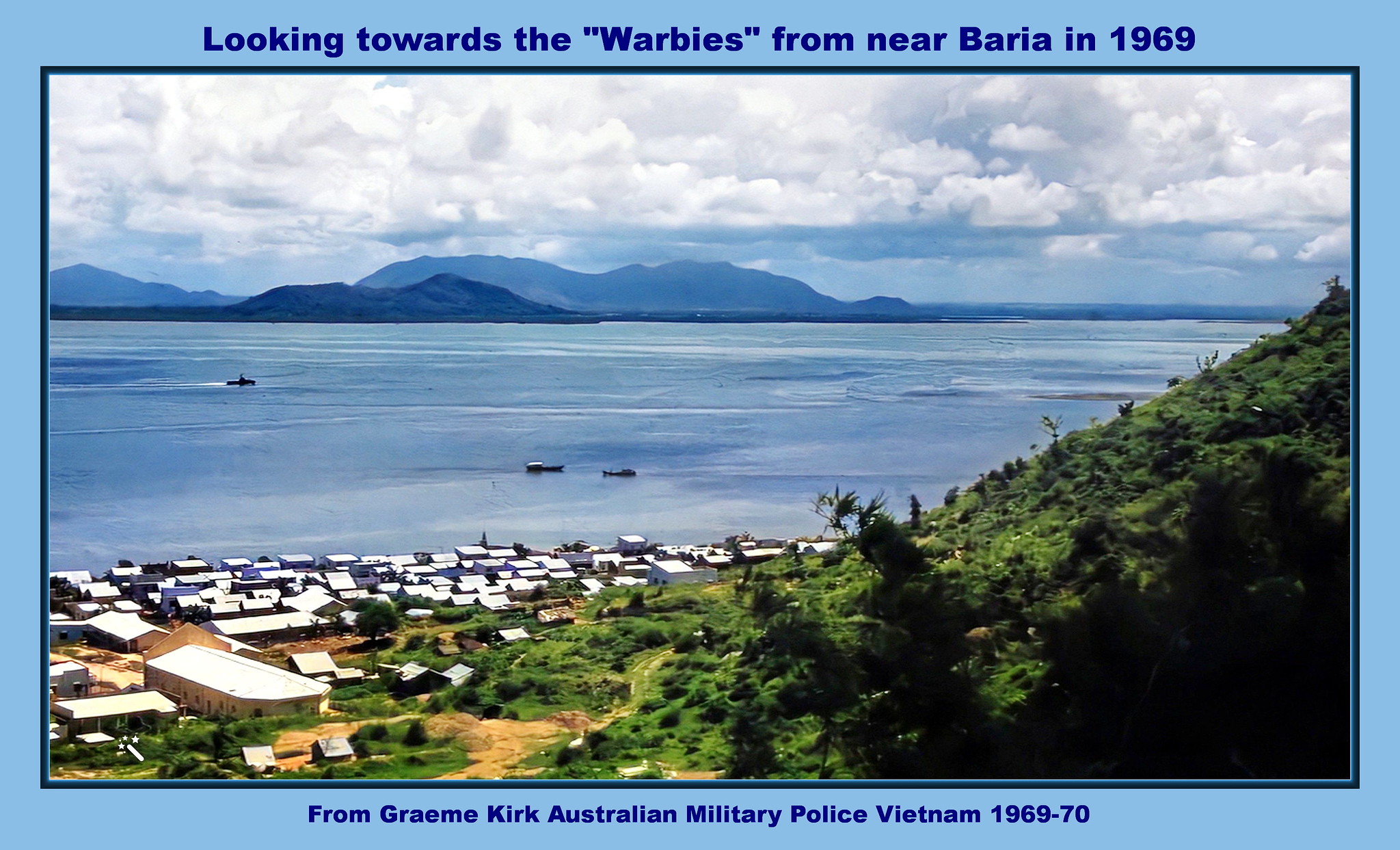The image is a photograph of an old postcard, surrounded by a light blue frame. At the top, the text reads "Looking towards the Warby's from near Baria in 1969," with "Warby's" in quotation marks and spelled as W-A-R-B-I-E-S. Below the photo, it says "From Graeme Kirk, Australian Military Police, Vietnam 1969-70."

The scene depicted in the postcard features a calm expanse of blue water stretching across the middle of the image, dotted with three visible boats: two in the center and one towards the left. In the near background stands a short, green mountain range, giving way to a higher, more distant mountain range. Fluffy cumulus clouds scatter across the sky, adding depth to the background.

To the right of the image, a green hill slopes gently down to the water’s edge, leading the viewer’s eyes to a collection of buildings along the shore. These buildings have white roofs—some flat, others with more traditional angles—indicating a small settlement. The setting, calm and picturesque, appears to be a large river or bay, framed meticulously to capture both the natural and man-made elements in harmonious balance.